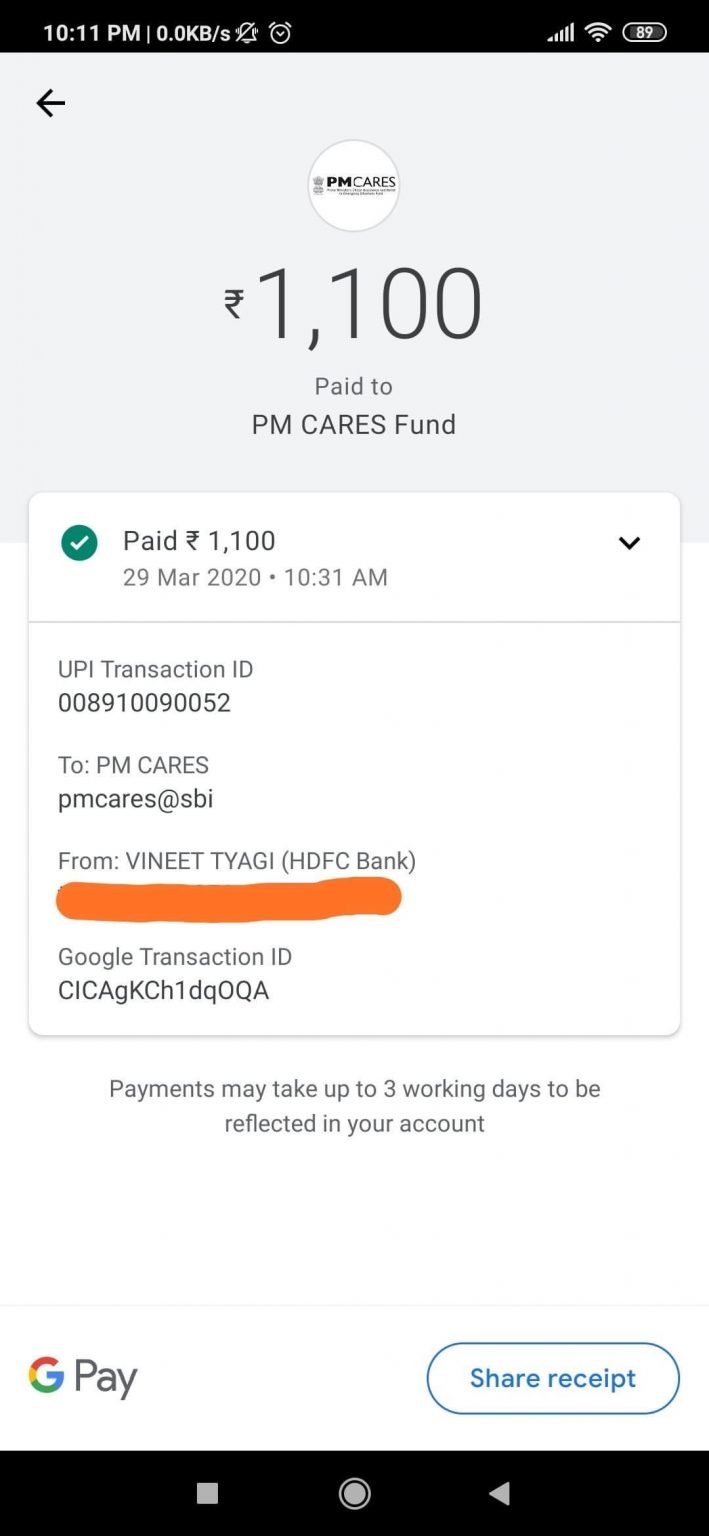This is a detailed screenshot of a smartphone displaying a transaction receipt. At the top of the screen, the time is shown as 10:11 p.m., with a data transfer rate of 0.0 KB/s. Accompanying this are several status icons, including symbols for an alarm, internet connectivity, and battery charge.

Beneath this is a gray header bar featuring a black arrow pointing to the left in the upper left corner. Central to this section, a figure of 1,100 is prominently displayed. To the left of this number is a unique monetary symbol resembling an "L" with two lines at the top.

Above this gray area, there is a circular icon containing a brand name that appears to be "PM CARES." Below the figure of 1,100, the text reads "Paid to PM CARES Fund."

Another section beneath this displays a white box with the word "Paid" and the monetary value symbol followed by 1,100. This is followed by a date and time stamp: "29 MAR 2020" and "10:31 a.m."

To the left of this section, a circle with a checkmark signifies that the transaction has been completed. To the right, a downward-pointing caret indicates an expandable dropdown menu, which has been opened in this screenshot.

Within this dropdown, details of the "UPI Transaction ID" are provided, followed by a string of numbers. Below this, it states "To: PM CARES (pmcares@sbi)" and "From: Vineet Tyagi (HDFC Bank)."

A portion of the screenshot shows a section marked off with yellow highlights, obscuring personal information. Lastly, there is a "Google Transaction ID" listing another string of letters and numbers.

A disclaimer notes that "Payments may take up to three working days to be reflected in your account." At the bottom of the screenshot, the icons for GPA and a "Share Receipt" bar are visible, alongside familiar phone iconography.